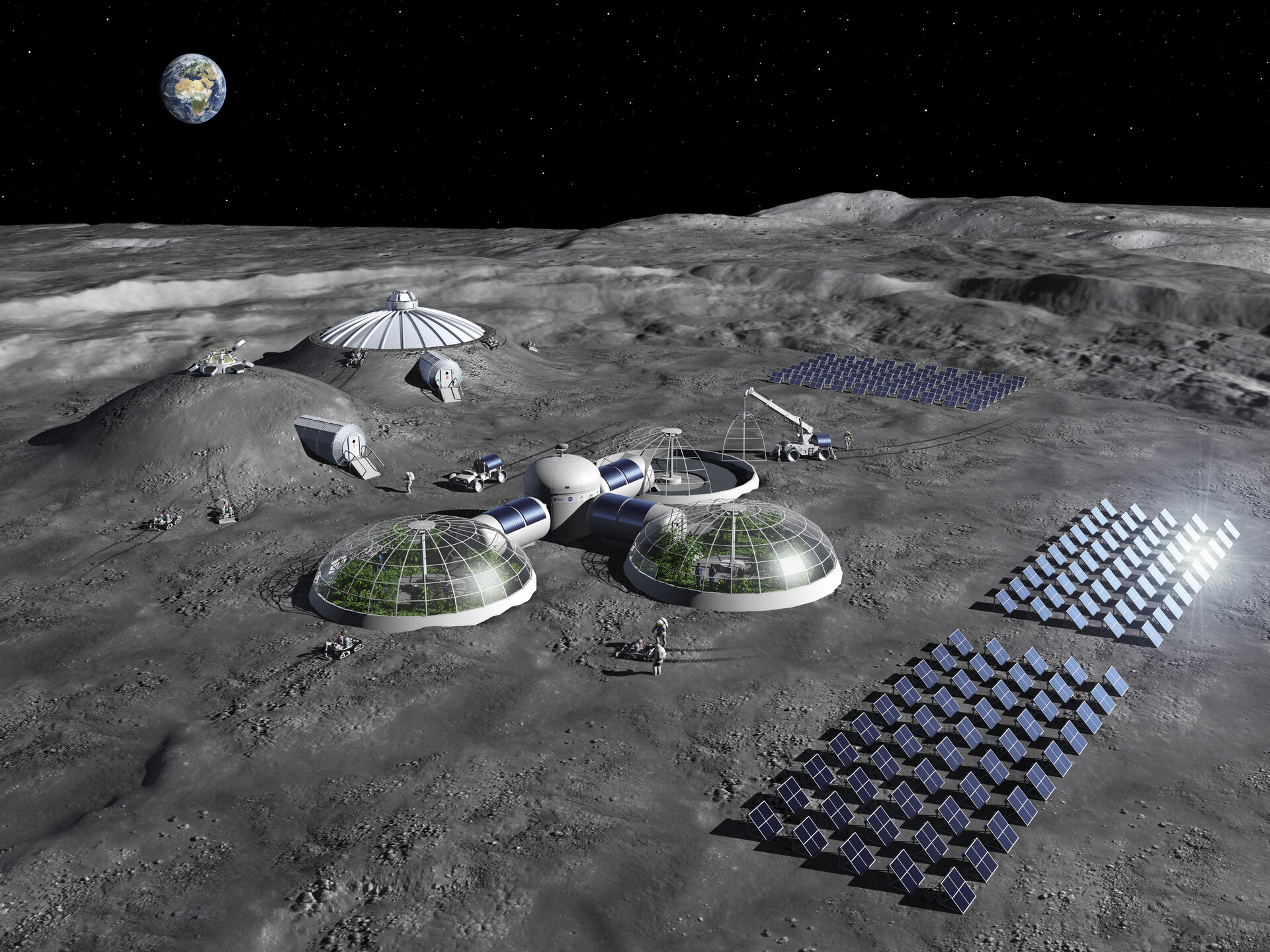This digital rendering depicts a lunar colony set against the rugged, light and dark gray landscape of the moon, with Earth visible in the distance and a star-filled black sky above. The colony consists of three interconnected biosphere domes radiating from a central hub, designed to sustain life by growing plants for oxygen and food. Two of these domes are fully constructed, housing visible greenery, while the third appears to be under construction. Additionally, another ecosystem section is built into the existing ground, showing only rooftops and entryways.

A vast array of solar panels, totaling between 20 and 40 units, is strategically placed around the colony to harness solar power. A solar panel on the right side and another on the top center of the image catch lens flares, indicating their operation under sunlight. An astronaut in a white suit can be seen working near the central hub, emphasizing ongoing construction and maintenance efforts for the colony. A vehicle is also present on a nearby mound, adding to the scene's sense of development and activity.